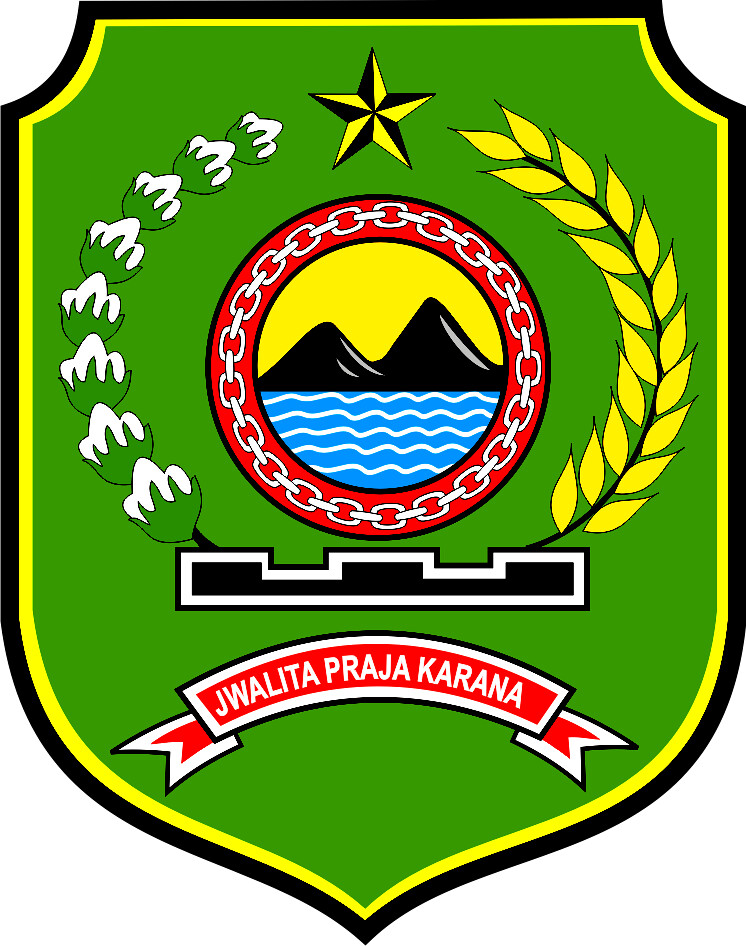The image depicts a computer-generated crest with a distinctive black border accented by a slim yellow stripe just inside the edge. The main body of the crest is a solid green color. At the very top center sits a yellow star shaded with black along some of its points. To the left of the star, green flowers with white tips arc gracefully downward in a chain-like formation. On the right, a black branch adorned with yellow leaves mirrors this curvature. Both the flowers and the branch form a border around a central circular emblem.

This emblem features an intricate design: a black circle outlined with an inner red stripe, which itself is bordered by another black line. The red stripe is decorated with a white chain that circles around the entire circumference. Inside the circle, a tranquil landscape is depicted, including a yellow sky, two black mountains, and blue water with white waves.

Beneath this emblem is a black-and-white outlined building that extends horizontally, with taller segments at the left, right, and center. At the very bottom of the crest is a white banner that curves outwards and then tapers back in, inscribed with "JWALITA PRAJA KARANA" in bold white letters against a red background.